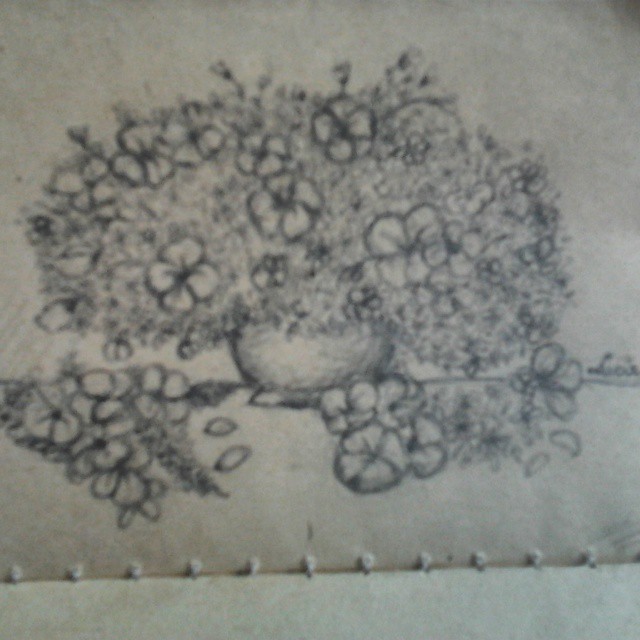A detailed pencil sketch captures a round vase or bowl overflowing with an abundance of flowers. The blossoms spill over the edges, cascading gracefully around the sides and front of the vessel. The artwork is meticulously drawn on a light-colored piece of parchment paper, enhancing its vintage charm. Below the main sketch, a secondary layer of paper or fabric is visible, adorned with evenly spaced, small round threads, adding an extra layer of texture to the composition. The overall quality of the image appears slightly out of focus, lending a soft, blurred effect to the intricate details of the drawing.